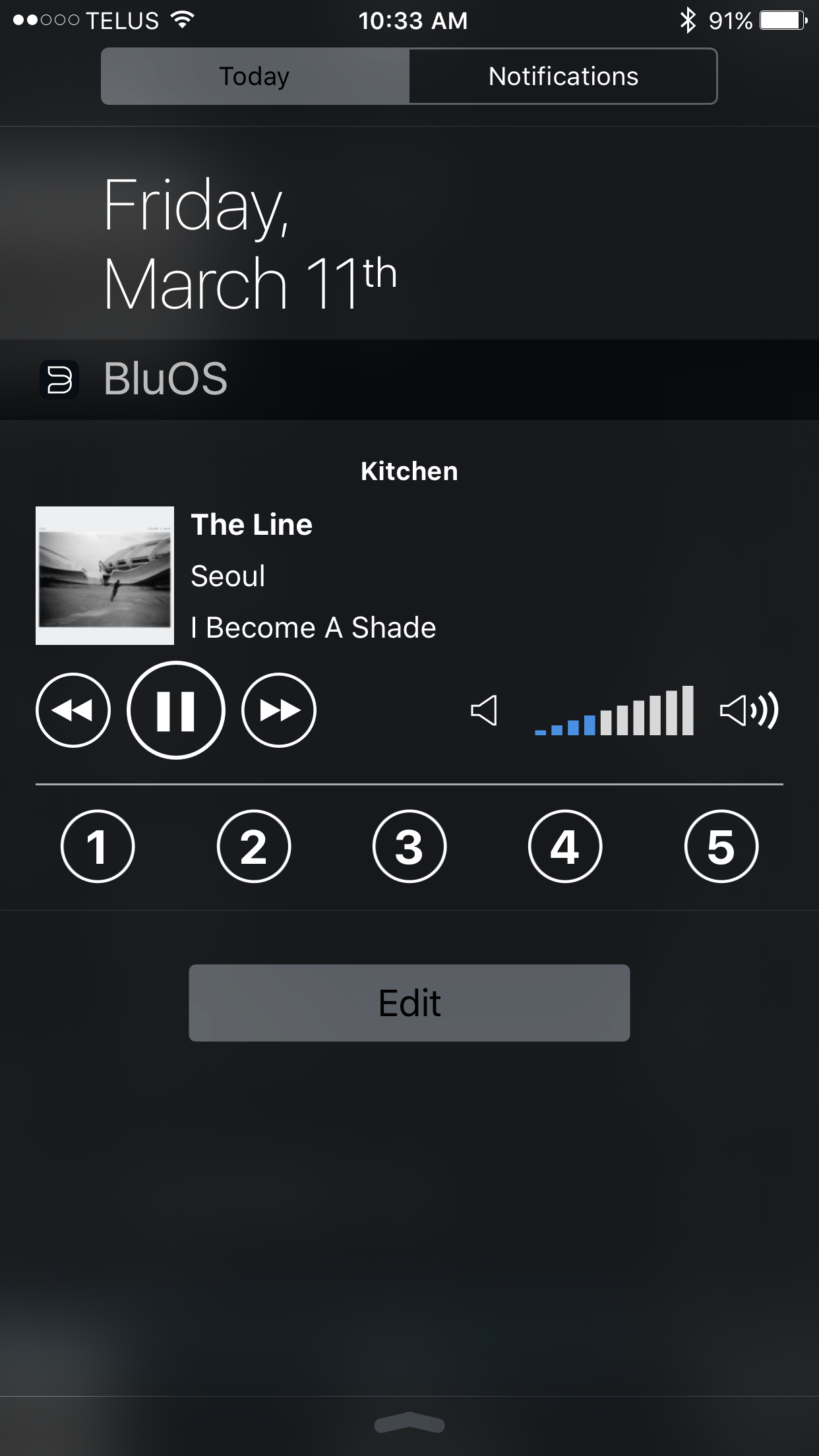The image displays a smartphone screen against a black background, featuring several interface elements. At the top, the screen shows the time as 10:33 AM, the carrier as TELUS, a battery indicator at 91%, and a Bluetooth symbol. Below this, two primary rectangles are visible: a gray one with "Today" written in black, and a black one with "Notifications" written in white. The date is highlighted as Friday, March 11th.

In the main section of the screen, there appears to be an operating system interface, indicated by "BOS" in capital letters, colored blue. The interface mentions "kitchen" and displays a photo of two people water skiing, with a caption or label possibly related to "lawn seal." 

Overlaying the image are media control buttons, including a pause button, a play button, and a rewind button, as well as a speakerphone icon and a speakerphone icon with three signal bars.

There are several rectangles, with the first four shaded blue, and possibly some other shapes that may not be rectangles. Additionally, there are numerical indicators from one to five inside circles. Below the main area, there’s a gray rectangle labeled “Edit” in black text. At the very bottom center of the screen, there is an arrow pointing upward.